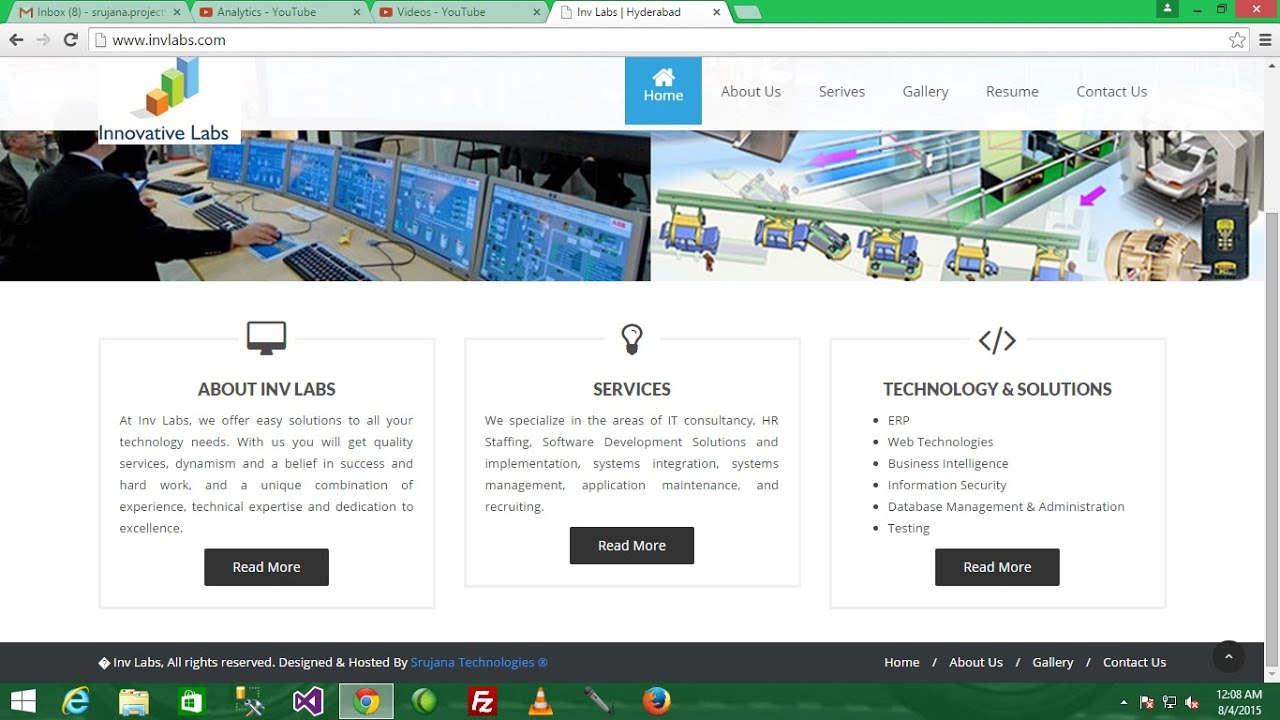This image displays a screenshot of a web page loaded on a computer, with the taskbar icons clearly visible at the bottom, suggesting it is on a Windows operating system. At the very top, the browser's interface is visible with multiple open tabs, including Google Mail, YouTube, and analytics tools, indicating active user sessions. Below the tabs, the URL in the address bar points to "www.invalabs.com," the website for Innovative Labs.

The website features a green header and a navigation bar with links to "Home," "About Us," "Gallery," "Resume," and "Contact Us." Two prominent illustrations are displayed on the page: one of a man surrounded by computer monitors, and another showcasing a car production line. Below these images, there are three content boxes:

1. **About INV Labs:** This section includes a "Read More" button for additional information.
2. **Services:** Outlines what the company specializes in, with a "Read More" button.
3. **Technology and Solutions:** Lists key areas such as ERP, business intelligence, and information security, accompanied by bullet points.

The bottom edge of the screenshot shows the typical taskbar icons, rounding out the interface view.